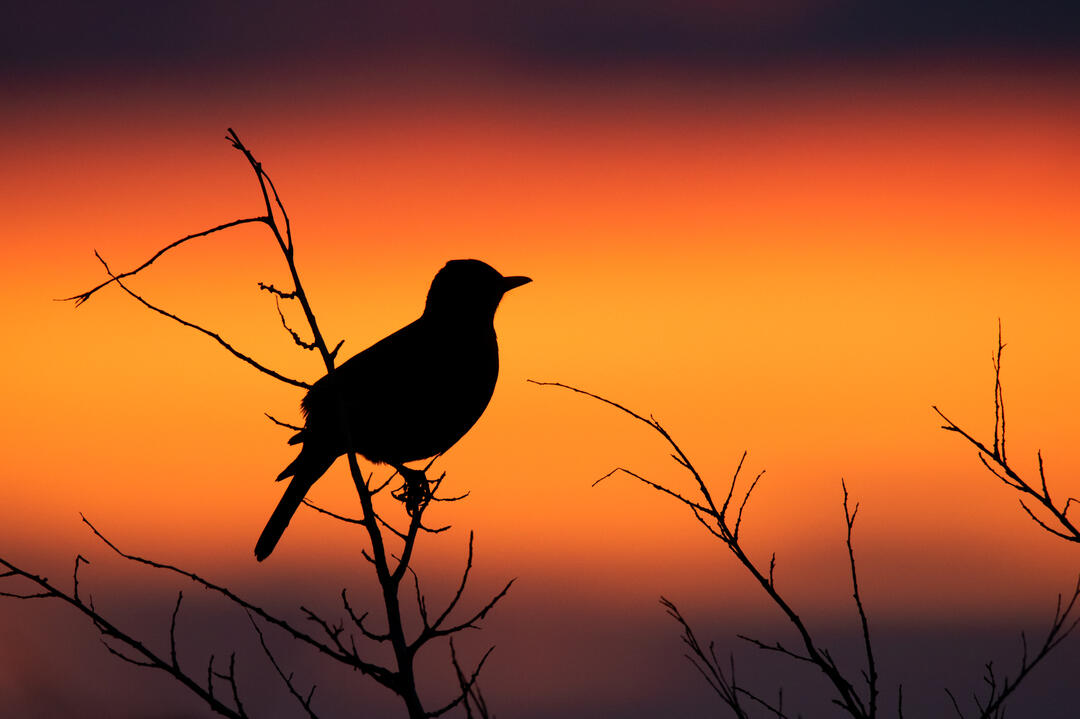This horizontal color photograph captures a serene twilight scene, where the deep orange, red, and dark yellow hues of the sky create a muted, enchanting backdrop signaling the end of the day. The silhouette of a small bird, potentially resembling a chickadee, is perched elegantly on one of the highest, thin, leafless branches on the left side of the image. The bird, entirely in shadow yet intricately defined with a clear beak, tail, feathers, legs, and claws, faces to the right, seemingly bidding farewell to the day and welcoming the approaching night. The dark outlines of the branches and the small bird against the ambient glow of the transitioning sky enhance the peaceful, contemplative mood of the image.